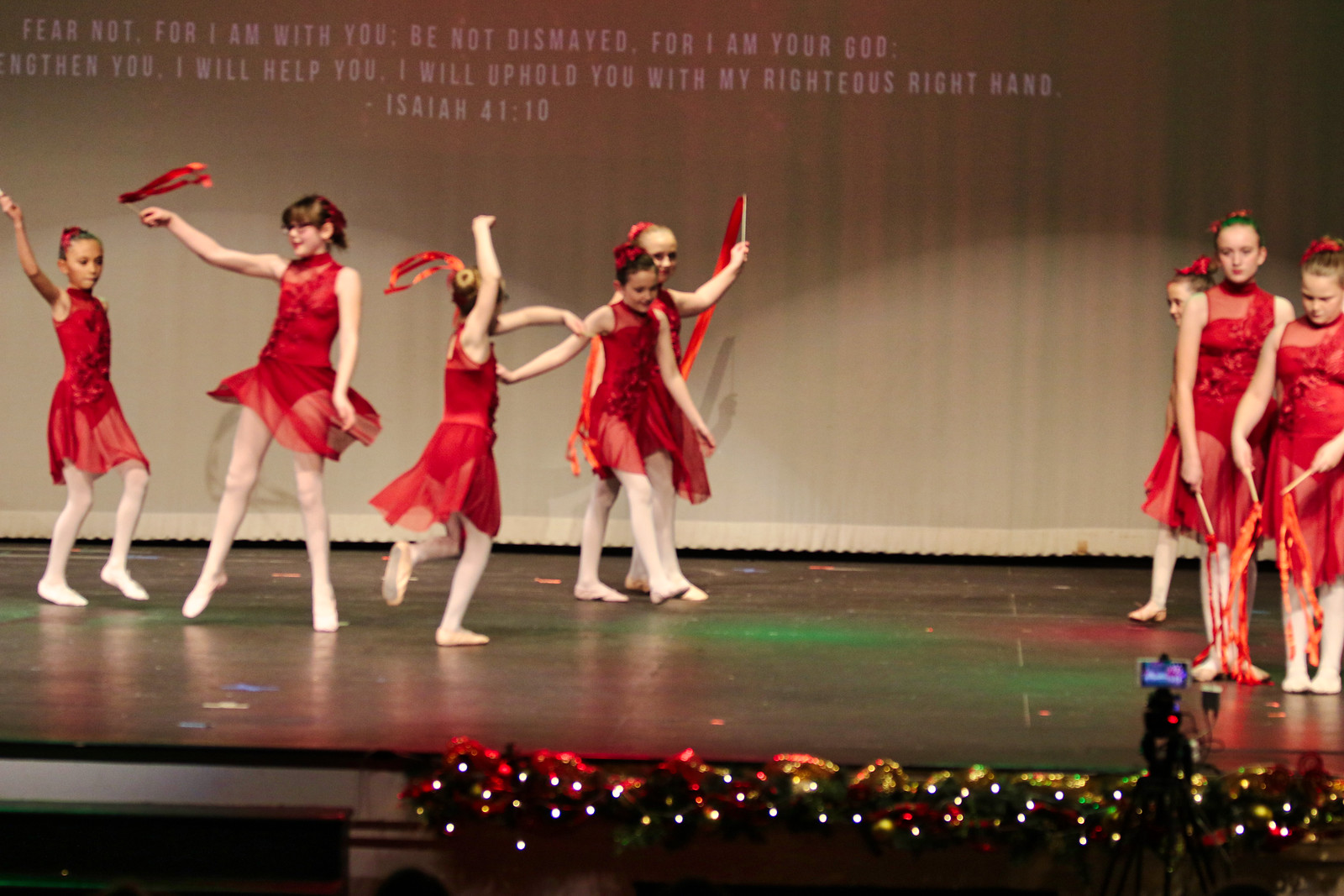The scene depicts a color photograph in landscape orientation of a vibrant Christmas show. The stage is adorned with festive red, green, and white lighted decorations, evoking a holiday atmosphere. Centered on the dimly lit stage are eight young girls performing a coordinated dance. They are dressed in matching red outfits featuring red leotards, sheer red skirts, and white stockings. Each girl wields a stick with red sashes or banners, which they wave gracefully as part of their routine. 

The stage's backdrop features a beige curtain with a projected Biblical verse in white text, stating: "Fear not, for I am with you; be not dismayed, for I am your God. I will strengthen you, I will help you, I will uphold you with my righteous right hand. – Isaiah 41:10." The girls' hair is tied back, appearing short to avoid interference with their performance. In the foreground, delicate white twinkle lights border the stage, adding to the festive ambiance. A tripod with a camera is visible, capturing the event, underscoring the lively, participatory nature of the celebration.